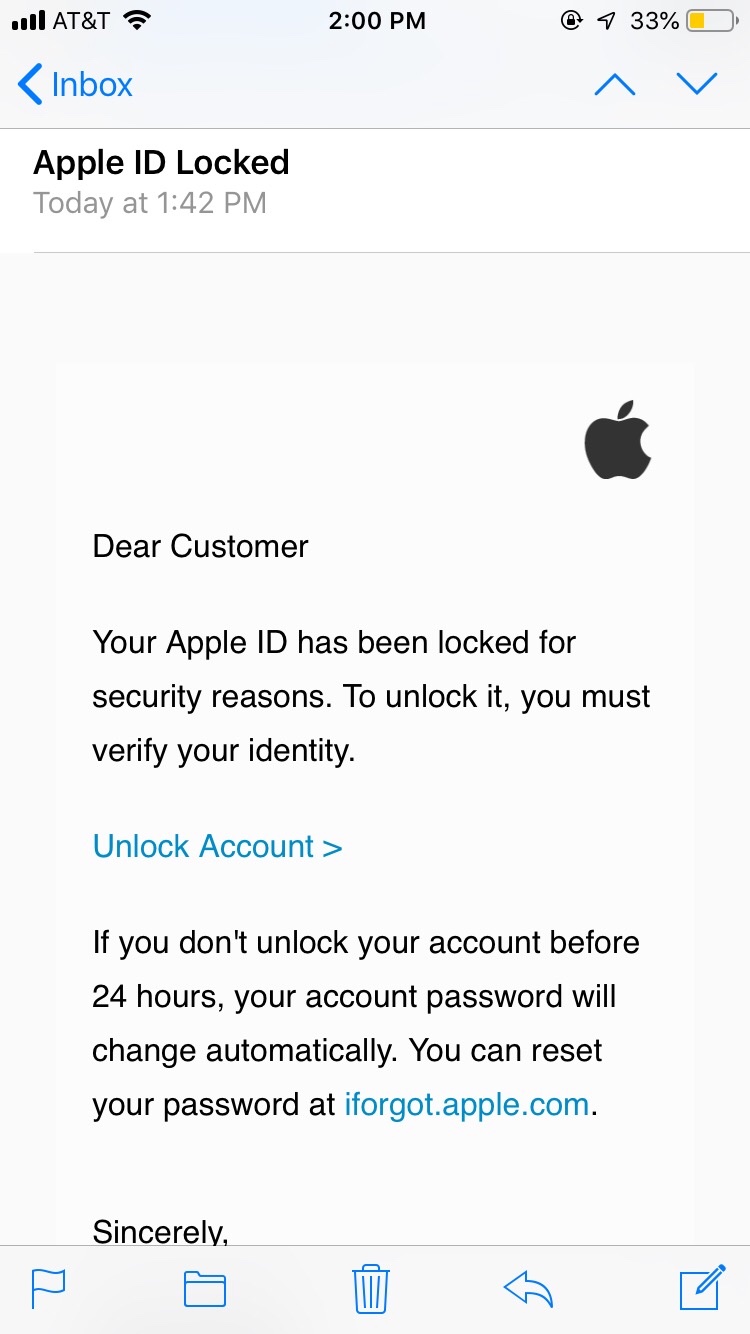Detailed Caption:

Displayed on an iPhone screen, there is an email from Apple notifying the user of a security issue. The top of the screen shows full cellular bars for AT&T, active Wi-Fi, and the time reading 2:00 p.m. Various status icons include an airplane mode indicator and a 33% battery level depicted in yellow. The email interface, marked by a blue-tinted 'Inbox' header with a back arrow, reveals an email below with the subject line "Apple ID Locked."

The email reads, "Dear customer, your Apple ID has been locked for security reasons. To unlock it, you must verify your identity." A blue hyperlink labeled "Unlock Account" with an arrow is provided. The message warns, "If you don't unlock your account within 24 hours, your account password will change automatically. Go set your password at Iforgot.Apple.com."

The signature line ends abruptly with "Sincerely" followed by a visual cut-off. At the bottom of the email interface, there are options to flag, trash, reply, forward, or archive the email, represented by blue icons for each action: a flag, folder, trash can, back arrow, and a pencil writing on paper. Given the context and appearance, this email appears to be either a phishing attempt or a legitimate alert that the user's Apple ID has been locked for security purposes.